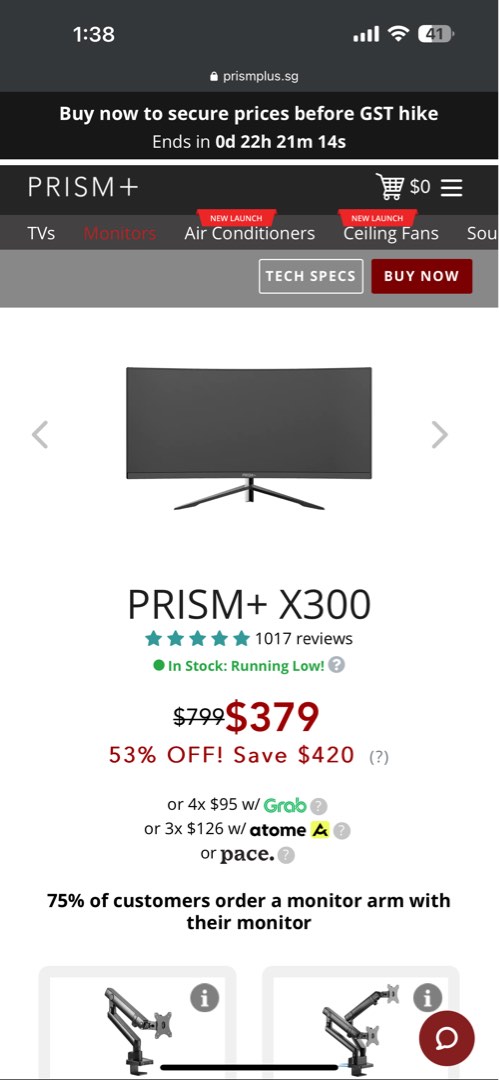Screenshot Details:

- **Background**: White
- **Time Displayed**: 1:38
- **Battery Level**: 41%
- **Website Prompt**: "Buy Now to Secure Prices for GST" (likely relating to a price hike)
- **Countdown Timer**: 0 Days, 22 Hours, 21 Minutes, 14 Seconds remaining

Website Elements:
- **Website Name**: Prism+ (all in capital letters)
- **Shopping Cart**: Displays "$0"
- **Navigation Menu**: Hamburger icon
  - Categories: TVs, Monitors, Air Conditioners, Ceiling Fans

Product Information:
- **Category**: Monitor
- **Model**: Prism+ X300
- **Rating**: 5 stars from 1,017 reviews
- **Stock Status**: "In Stock - Running Low" indicated by a green circle
- **Price**: 
  - Original: $799 (crossed out)
  - Discounted: $379 (in red)
  - Percent Discount: 53% off
  - Savings: $420
- **Additional Purchase Option**: "$95 x 4" (payment plan) with a "W/GRAB" (indicating use of a specific payment method, displayed in green)

**Note**: Additional symbols and notations include a question mark in a gray circle, indicating further information or assistance is available.

Descriptive Caption:
"A screenshot from an e-commerce website at 1:38 with 41% battery level showcases a promotional deal on the Prism+ X300 monitor. The site encourages users to 'Buy Now to Secure Prices for GST' with a countdown timer showing 22 hours, 21 minutes, and 14 seconds remaining. The user interface includes a shopping cart icon indicating a $0 balance and a hamburger menu linking to various product categories like TVs, Monitors, Air Conditioners, and Ceiling Fans. The focus is on a Prism+ X300 monitor rated 5 stars by 1,017 reviews, which is 'In Stock - Running Low' as shown by a green circle. The monitor's price is slashed from $799 to $379, a 53% discount saving users $420. An additional purchase option offers four installments of $95 through 'W/GRAB.' Additional help is available, as indicated by a question mark in a gray circle."